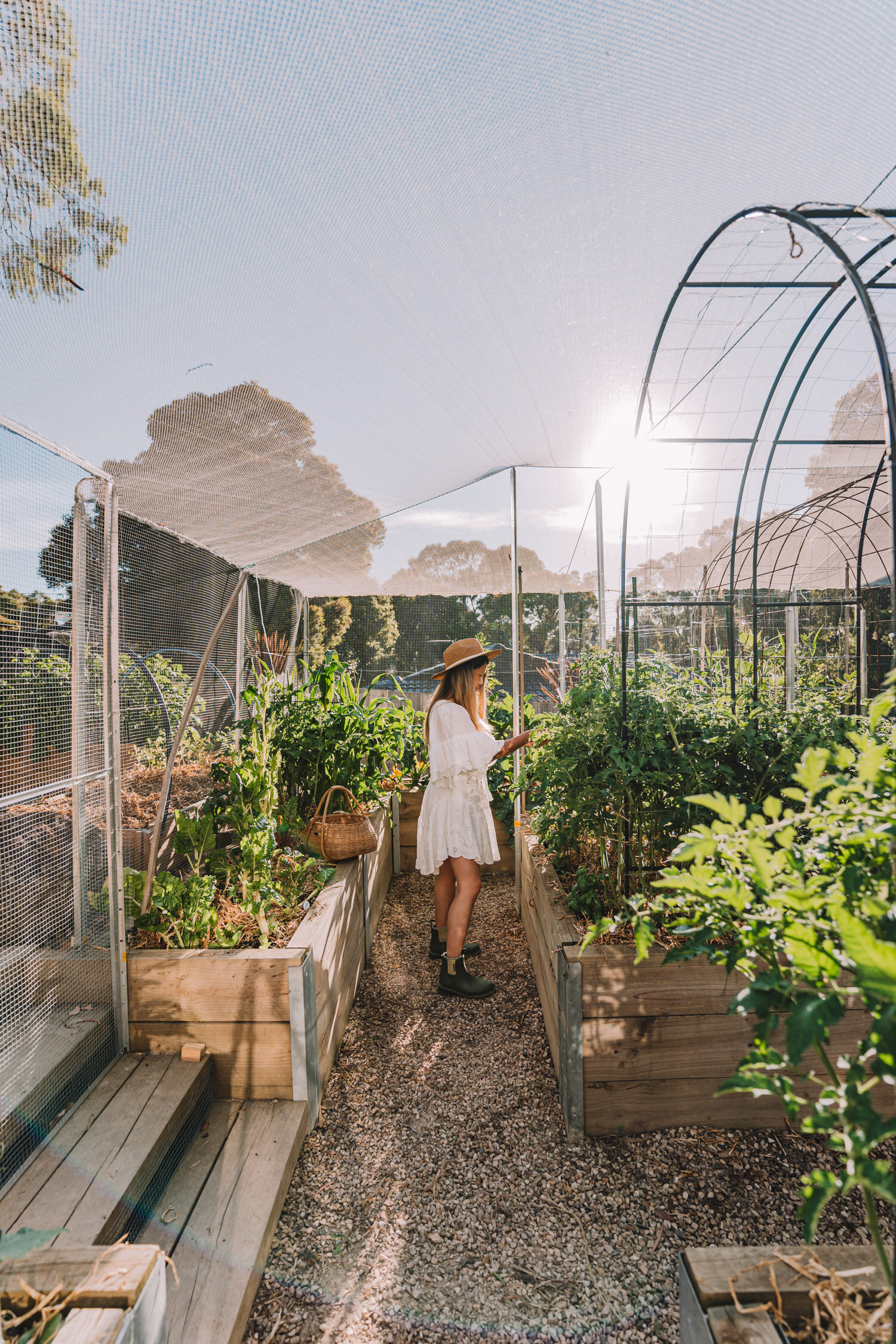In this captivating daytime outdoor photograph, we see a garden center or outdoor greenhouse bathed in sunlight, indicated by the bright sun visible at the back of the image. The central focus is a young woman with long, possibly blonde hair, wearing a wide-brimmed straw hat and a short, flowy white lace dress that ends above her knees, paired with short black ankle boots. She stands midway between two wooden flowerbeds, filled with various green plants, some adorned with small white flowers. A wicker basket rests on the ledge of one flowerbed behind her. To the right, a green metal archway, covered with vines, stands prominently. The rocky path beneath her feet extends straight back and curves to the right, leading to a short set of stairs visible in the bottom left corner. The entire garden area is enclosed in protective netting, adding structure to the serene scene, accentuated by the fence surrounding the perimeter.